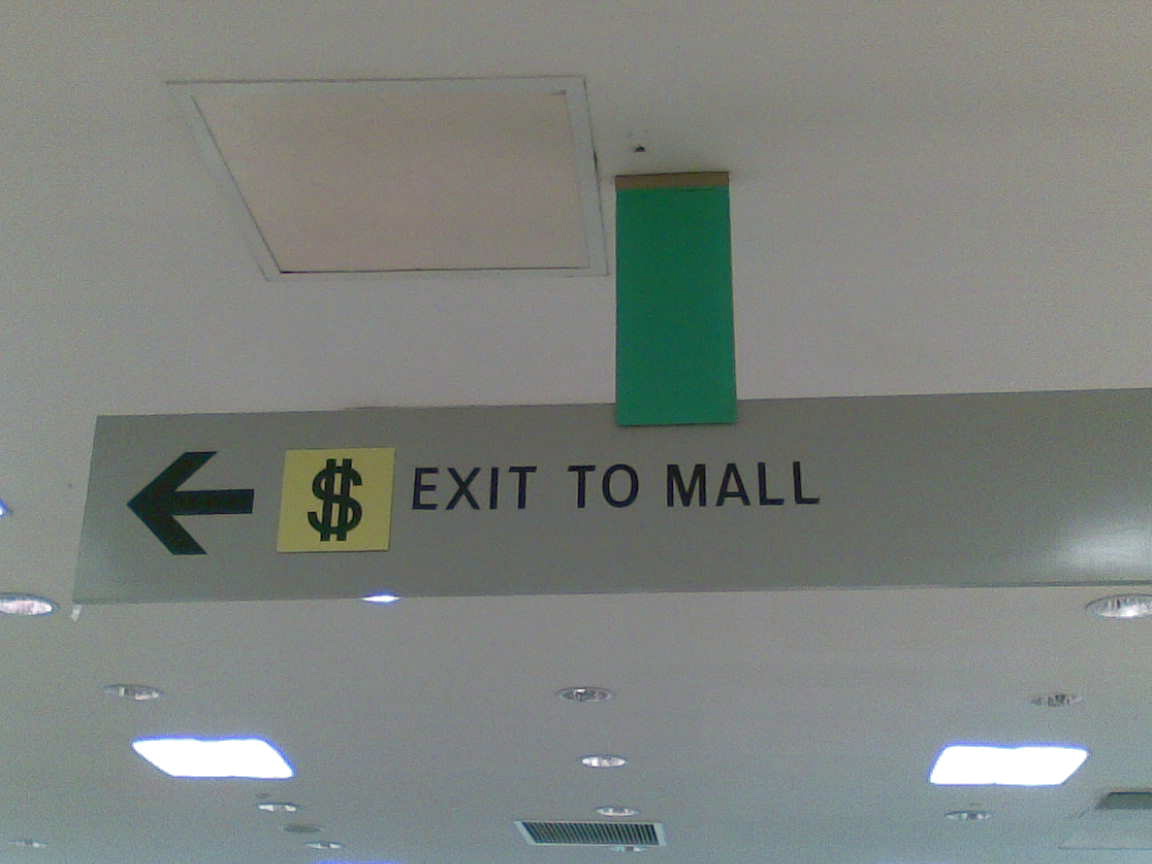This photograph captures the interior ceiling of a building, focusing on a hanging sign that provides directional instructions. The rectangular sign features the words "EXIT TO MALL" in prominent black lettering. To the left of the word "EXIT," there is a graphic of a dollar sign ($) set against a yellow square background. Adjacent to this dollar sign, an arrow points leftwards, directing off-screen. The sign is affixed to the ceiling by a vertically rectangular green support bar, which connects it sturdily to the ceiling. Above, the ceiling appears standard, painted white, with evenly spaced lighting fixtures illuminating the area. The overall composition of the image provides a clear indication of the exit route toward the mall, enhanced by the straightforward yet informative signage.